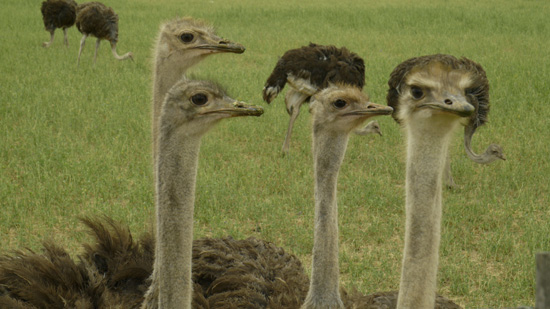The photograph features a group of eight ostriches in a grassy green field, capturing the essence of the natural habitat of these fascinating birds. In the foreground, four ostriches dominate the center of the image, their heads and elongated necks standing out prominently. They exhibit a striking contrast in coloration, with tan heads and necks transitioning into darker, fluffier brown bodies. Most of these ostriches seem to be gazing towards the right, with one slightly directing its attention more towards the viewer.

Towards the back of the field, more ostriches can be seen, although their heads are lowered, possibly grazing. Two of them are situated on the right, partially obscured by the nearer birds, whereas another pair is positioned in the far-left corner, making their exact orientation a bit challenging to discern. One notable detail is the unique ‘hairdo’ of one ostrich, featuring a crown of feathers that are somewhat different from the rest, adding an amusing and distinctive element to the scene.

The grass in the field varies in height and color, with patches of brown soil visible through the green clusters. This setting, possibly an Australian habitat, provides a vivid backdrop for the ostriches' engaging and seemingly inquisitive demeanor. Overall, the photograph not only showcases the physical attributes of the ostriches but also invites viewers to delve deeper into the intriguing world of these majestic birds.